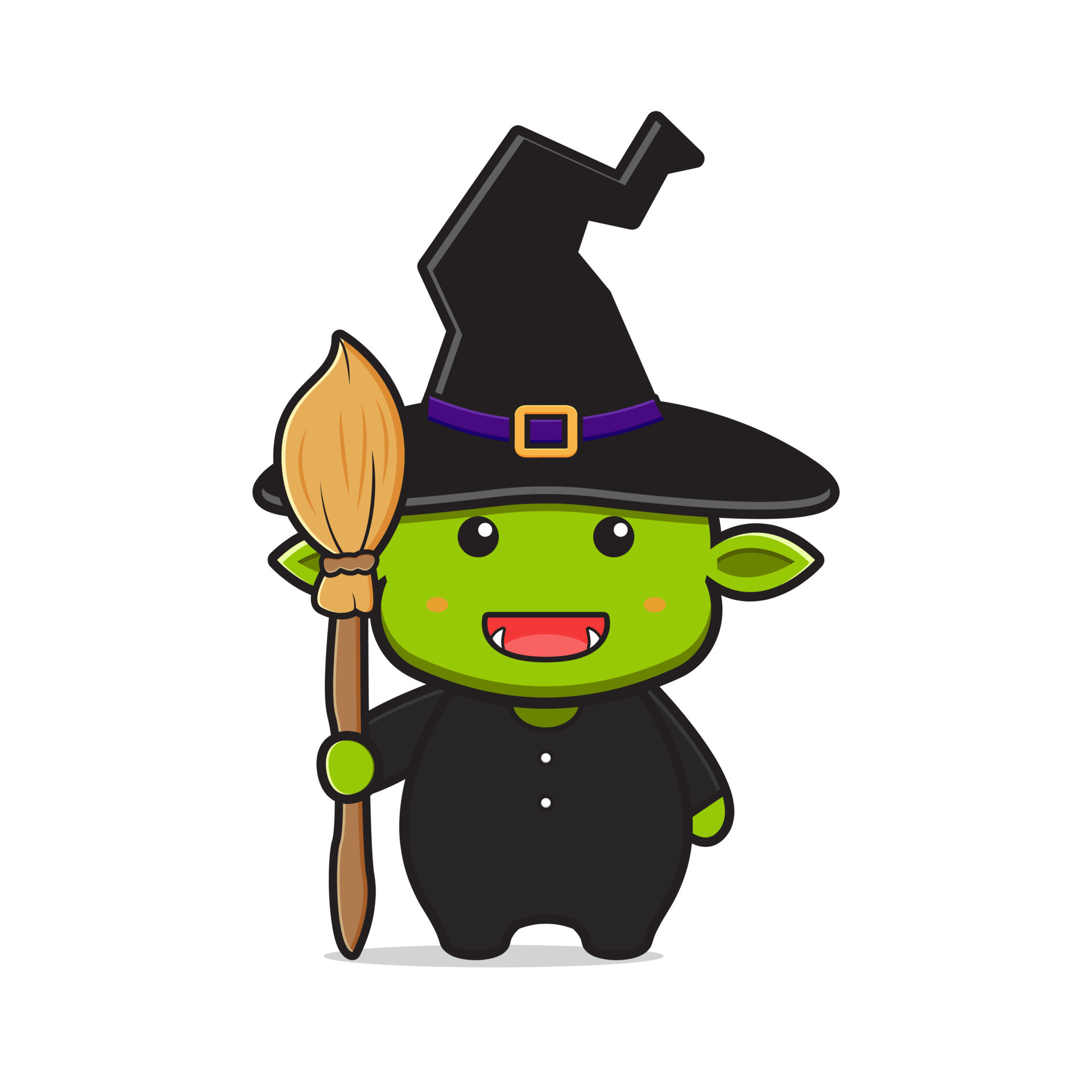The image is a detailed cartoon illustration of a small, green-skinned witch with pointy ears. She wears a large, crooked black hat adorned with a purple ribbon and a gold-colored square buckle in the center. Her playful expression features black, beady eyes with tiny white highlights and a mouth open in a smile, revealing two sharp, pointy teeth and pink dimples on her cheeks. She is dressed in a black jumpsuit with two white buttons on the chest and has little green hands visible. In her right hand, she holds an upside-down broom with a brown handle and tan bristles. The character combines traits of both a witch and a gremlin, making for a whimsical and enchanting image.